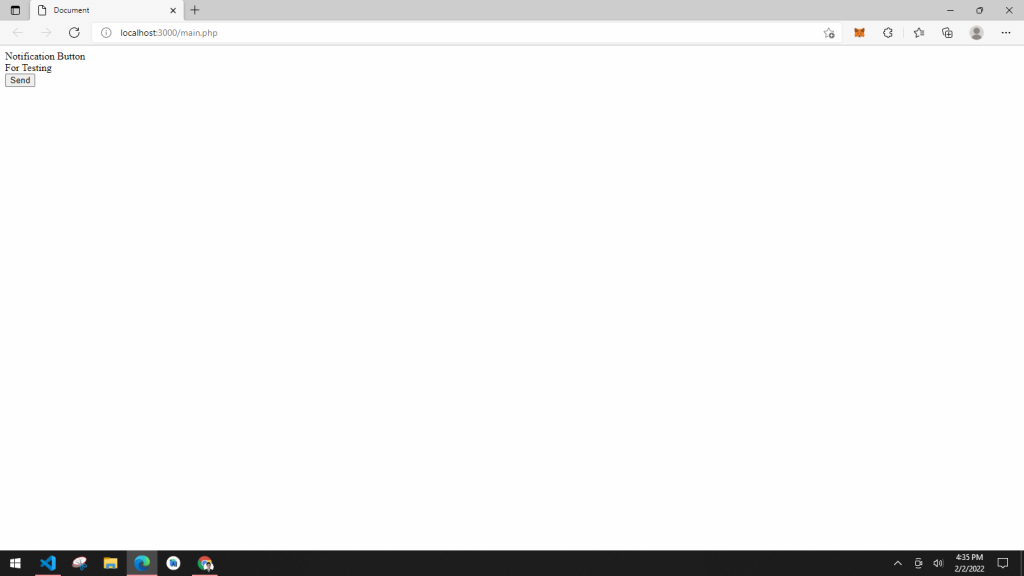The screenshot displays a computer screen featuring an open browser tab. In the upper left-hand corner, the tab is labeled "Document." On the far right side of the tab, visible icons include the minimize button, a button to change the display orientation, and the close button. Below the tab, the address bar reads "localhost:3000/main.php," with a favorite button and several symbols, including a grey profile icon, on the right side of the address bar.

Within the loaded webpage, there is simple text located in the upper left-hand corner stating, "Notification button for sending. For texting, testing." Directly beneath this text, a button labeled "Send" is present. The rest of the webpage is completely white, devoid of any additional content.

At the bottom of the screen, the Windows taskbar is visible, featuring the Windows logo on the left side. In the bottom right corner, the system clock displays the time as 4:35 PM and the date as February 20, 2022.